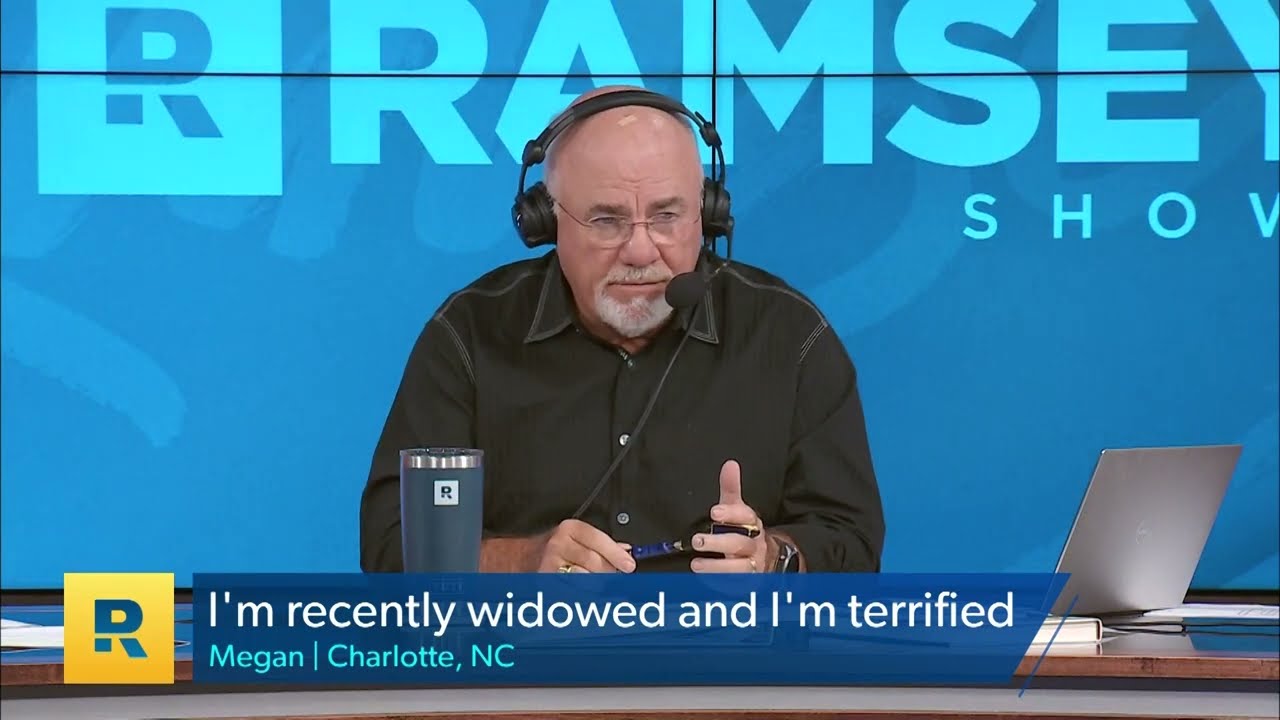A detailed screenshot captures an episode of The Ramsey Show, a call-in television program. At the center of the image sits an older white man, likely Ramsey, distinguished by his bald head, gray-white goatee, and small glasses. He wears a black button-up shirt and a black headset with an attached microphone. His intense expression suggests he is listening thoughtfully to the caller. Behind him, a grid of screens forms a blue digital backdrop, prominently displaying the RAMSEY SHOW logo in lighter blue text.

In front of Ramsey, a blue travel mug with an 'R' and an open laptop are visible. He holds a pen in his hands, indicating he might be taking notes. The chyron at the bottom of the image reads in white text, "I'm recently widowed and I'm terrified," and in blue text, "Megan, Charlotte, North Carolina." The Ramsey Show's gold square 'R' logo is also present in the lower left corner. The overall scene presents a detailed, engaged moment from a live call-in segment of the show.